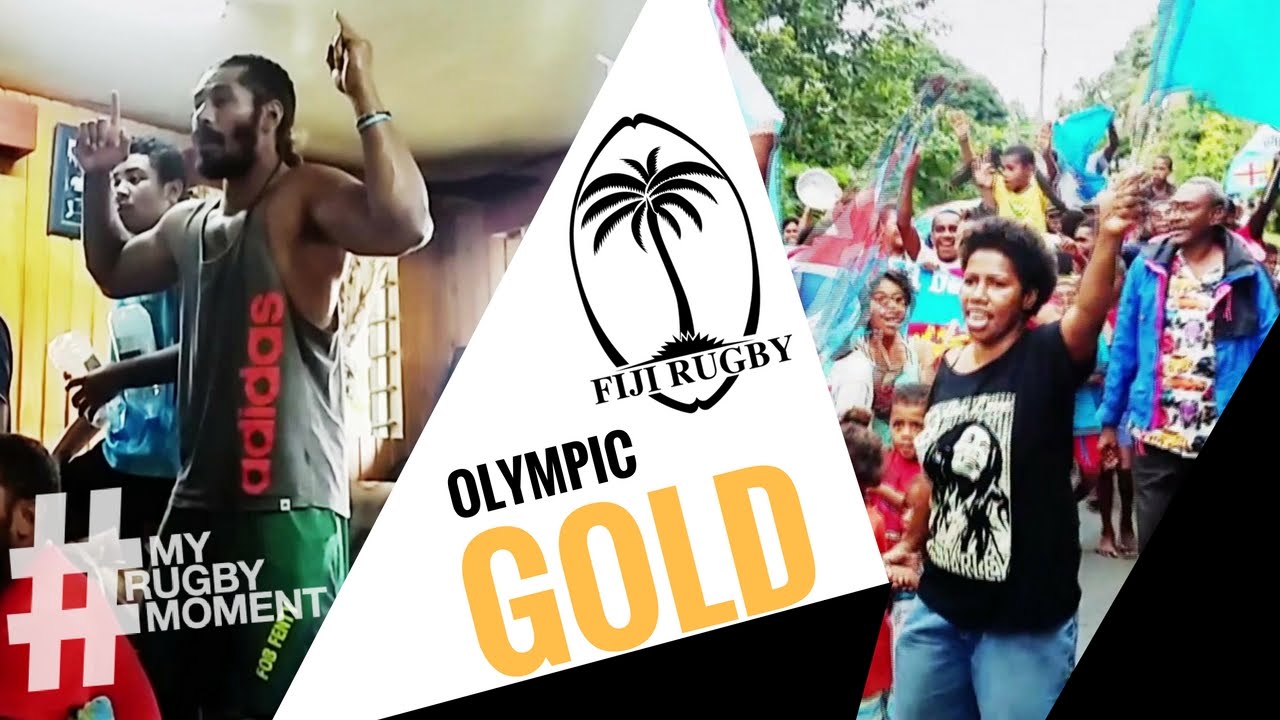This image appears to be a composite graphic advertisement for the Fiji rugby team, featuring two distinct photographs separated by a central logo. The logo, positioned in a skewed triangle, displays "Fiji Rugby" with a palm tree set inside an oval, likely symbolizing a coconut or surfboard shape. Below it, the words "Olympic Gold" are emblazoned in gold letters.

On the left side of the image, there is a man of African descent with a full beard, dressed in green shorts and a black Adidas tank top with "Adidas" in red letters on the front. His hands are raised beside his head, fingers pointed upwards, perhaps in a celebratory gesture. Standing next to him, there is a younger boy in a blue shirt and black pants, holding two water bottles. Superimposed over this portion of the image is the text "#MyRugbyMoment" in the bottom left corner.

The right side of the image showcases an outdoor scene with a diverse crowd of cheering fans. Most prominently, there is a Black woman wearing blue jeans and a black Bob Marley t-shirt featuring a white print of Marley's face and name. Her hand is extended upwards, joining others in the background who are also raising their hands in celebration. The crowd seems to be standing in a street setting with some foliage visible behind them, enhancing the festive atmosphere.